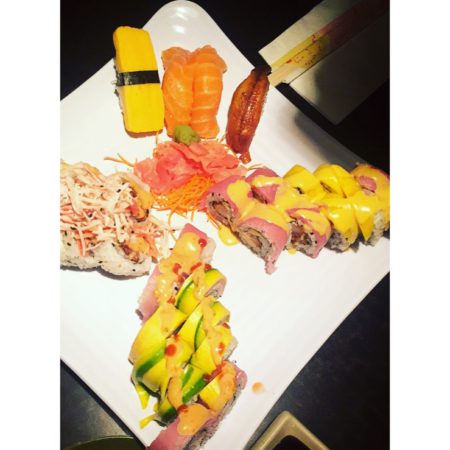In this detailed image taken inside what looks to be a fancy restaurant, we see a white square plate with rounded corners, positioned at a slight angle almost like a diamond, slightly off-center to the left. The plate is adorned with an artful array of sushi, creating a visually striking contrast with the black, white, yellow, orange, and pink elements present. 

At the top of the plate, there are three distinct pieces of fish sushi: a yellow rectangular piece, secured with a strip of dark green or black seaweed; two slices of salmon featuring characteristic lines on their surface; and a small brown fillet. 

In the very center of the plate, delicate, thinly layered pink pickled radish rests on a bed of shredded orange carrots, forming the central highlight. Arranged diagonally across the right side of the plate are pairs of circular sushi rolls, wrapped in pink and topped with a yellow sauce. At the bottom center, more sushi rolls appear in sets of two, featuring a combination of orange, yellow, and green sauces, adorned with shredded white and red meat atop rice.

Overall, the plate's diverse sushi selection and striking color palette create a harmonious and appealing presentation, emphasizing the care taken in its preparation and arrangement.